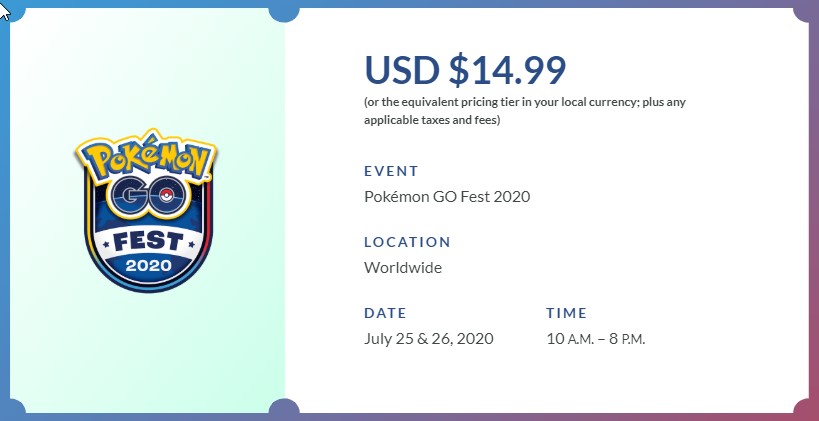This digital image is a screenshot of a transactional page for purchasing a virtual ticket to the Pokémon Go Fest 2020 event. On the left side of the image, there is a prominent green section featuring a badge that indicates "Pokémon Go Fest 2020."

On the right side of the image, the layout transitions to a white background with various text elements. At the top, there is a line of text in blue that reads "Enlarge," and directly beneath it, the ticket price is listed as "USD $14.99." The subsequent line clarifies that this pricing is subject to equivalent local currency rates and any associated taxes and fees.

Further down, the text continues to describe the event: "Pokémon Go Fest 2020." Following this, specific event details are highlighted in blue text. The location is noted as "worldwide," and the event dates are provided as "July 25 and 26, 2020," underscoring that it is a global virtual event spanning two days.